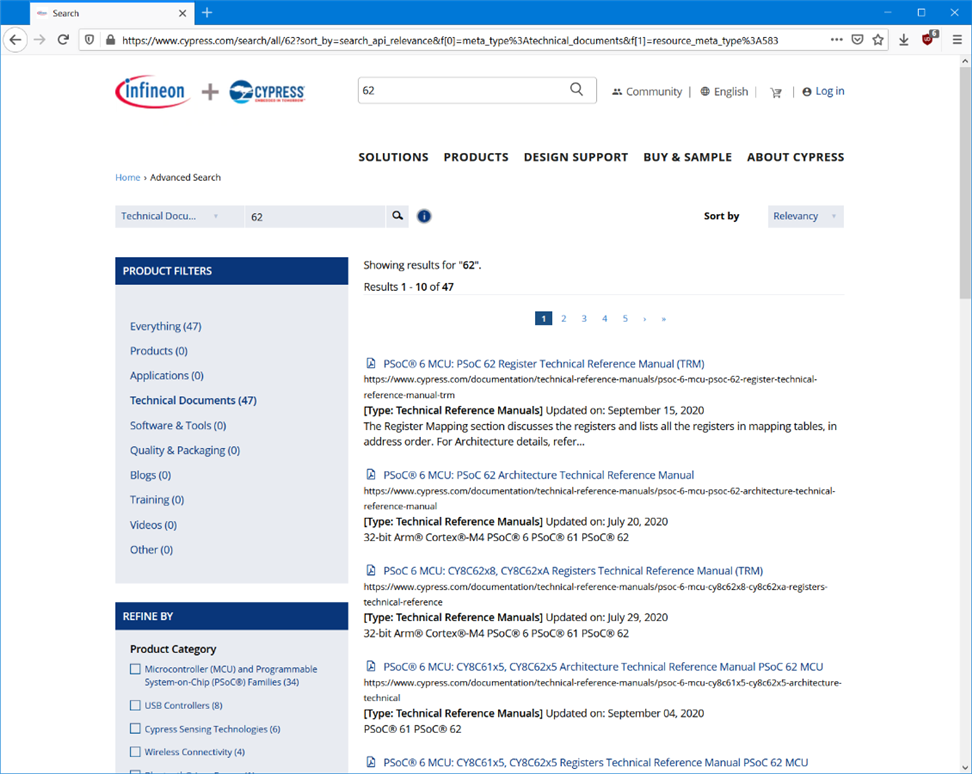The image is a screenshot of a Cypress Infineon's website, captured in a vertical rectangular format. The central focus is on a browser window showcasing the search box with the URL "www.cypress.com" followed by several backslashes. 

The top of the browser window is a bright blue bar. Moving down to the left side, the blue background continues but is interrupted by a small white search box at the top left corner, containing the word "Search" in black font.

Adjacent to the search box, slightly to the right from the top left corner, the word "Infineon" is prominently displayed in lowercase, bright blue letters. This text partially encircled by a red half-circle, excluding the letters "N-E-O-N." Next to "Infineon," a gray plus sign is visible along with a small circular logo that appears to be blue with white accents, though it is too diminutive to discern clearly. Further right, the word "Cypress" is printed in the same blue color with red lettering underneath.

The central area of the page contains several bold, black, all-caps headings: "SOLUTIONS," "PRODUCTS," "DESIGN SUPPORT," "BUY & SAMPLE," and "ABOUT CYPRESS."

On the left side of the webpage, under a navy blue horizontal box labeled "PRODUCT FILTERS" in white letters, a vertical light gray box lists filtering categories in navy blue font. The categories, each with parentheses enclosing item counts, include: "Everything (47)," "Products (0)," "Applications (0)," "Technical Documents (47)," "Software and Tools (0)," "Quality and Packaging (0)," "Blogs (0)," "Training (0)," "Video (0)," and "Other (0)."

Below this section is another navy blue horizontal rectangle labeled "REFINE BY" in white letters. Under this, "Product Category" is specified in bold black font against a gray background. Categories in blue font follow: "Microcontroller (MCU)" and "Programmable System on Chip" are partially visible, along with "USB Controllers (8)," and "Wireless Connectivity." Each category features an adjacent square checkbox, all unchecked.

The center of the image displays search results, albeit difficult to read. The first result seems to reference a technical manual.